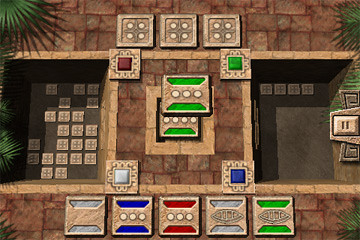This image showcases a vibrant screenshot from a tile-based puzzle game. The game board is framed by lush green vegetation in the top left-hand corner and along the sides, creating a visually appealing border. The central area features intricate tiles that the player likely has to match. On both the right and left sides of the gameplay area, there seem to be repositories for these matched tiles. At the bottom of the screen, several tiles are visible, each distinguished by colorful borders—white, blue, red, and green—and adorned with intricate designs or dots in the middle. The detailed artistry and thoughtful layout suggest a challenging and engaging puzzle experience.